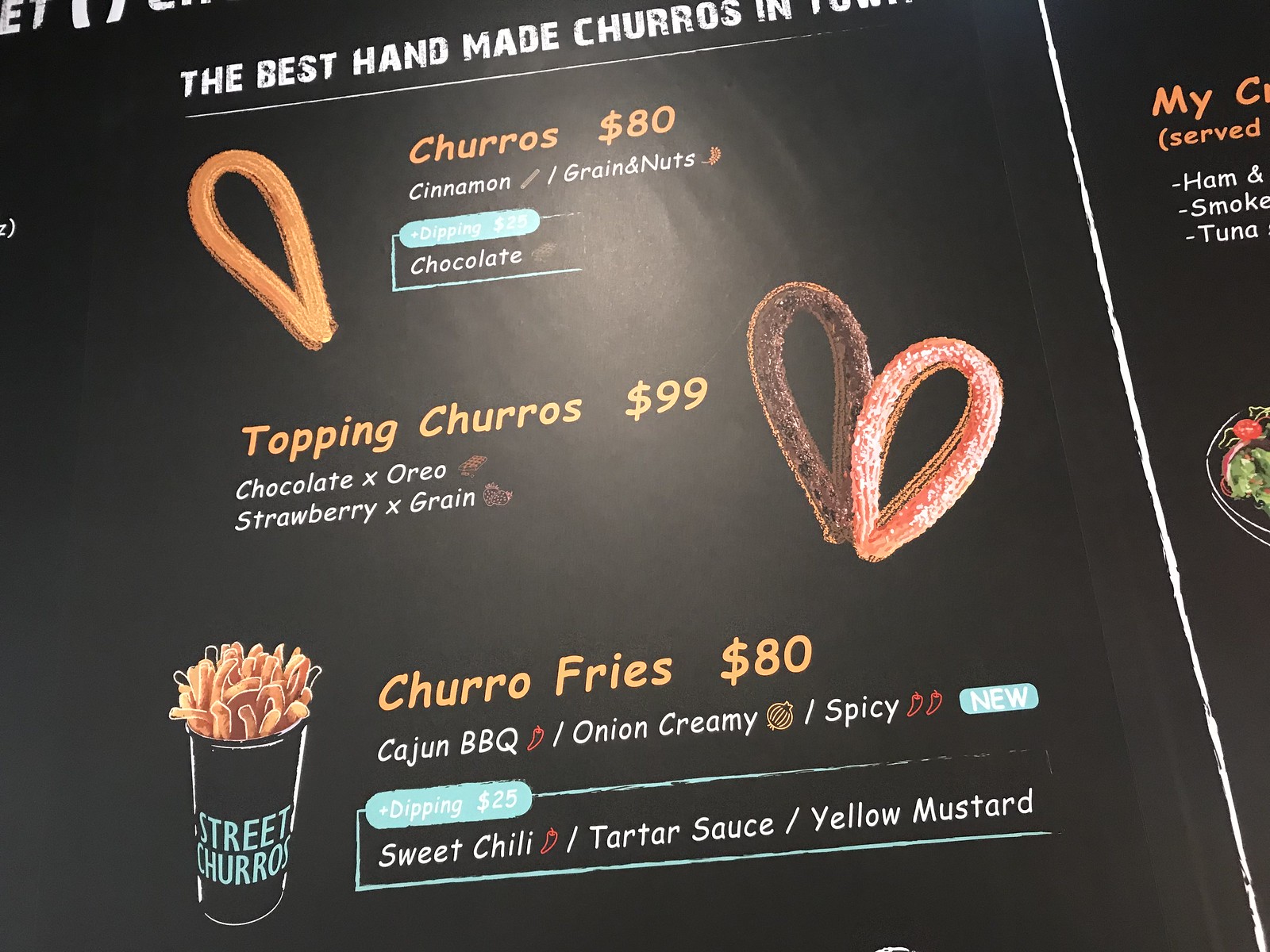This image showcases a section of a restaurant’s menu, presented on a black background with printed white text and illustrations, designed to resemble chalk writing. 

At the top, the menu proudly declares, "The Best Handmade Churros in Town." Below this announcement, there is an enticing image of a churro, alongside a price listing: "Churros - $80." The available flavors for these churros are "Cinnamon/Grain and Nuts," with dipping sauces offered for an additional $25, including a luxurious chocolate sauce.

Further down, the menu features "Topping Churros - $99," accompanied by an illustration of two churros positioned side-by-side to form a heart shape. These churros are available in two delectable combinations: "Chocolate X Oreo" and "Strawberry X Grain."

Beneath these options, the menu introduces "Churro Fries - $80," depicted adorably like French fries and served in a cup labeled "Street Churros." These churro fries can be seasoned with various flavors such as "Cajun BBQ," "Onion Creamy," and "Spicy"—which is touted as being twice as spicy as the Cajun BBQ and noted as a new addition.

Finally, a selection of dipping sauces for the churro fries is offered, including "Sweet Chili," "Tartar Sauce," and "Yellow Mustard," providing a diverse range of taste experiences to complement the churros.